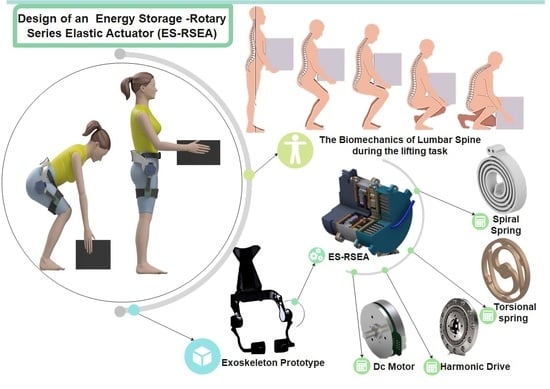The image is a detailed infographic showcasing the design and components of an Energy Storage Rotary Series Elastic Actuator (ES-RSEA). The background is completely white, with a mint green rectangle positioned at the top left corner containing the title "Design of an Energy Storage Rotary Series Elastic Actuator (ESRSEA)" in black font. Below this is a side-by-side comparison of a digitally rendered woman wearing a yellow shirt and light blue workout shorts, performing a lifting task. The sequence illustrates her biomechanical movement as she progressively bends down to pick up a black box and then stands back up, highlighting the proper spine alignment during the task.

To the right, there's a diagram resembling a silhouette in various stages of lifting a box, which is captioned "Biomechanics of Lumbar Spine During the Lifting Task." Beneath this are labeled components of the ES-RSEA, including a spiral spring, torsional spring, harmonic drive, DC motor, and an exoskeleton prototype. These elements form a semicircle around a central metal electrical part, which features a complex design with interconnected circles in blue, gray, dark gray, and brown. This detailed layout collectively illustrates the operational mechanics and construction of the ES-RSEA exoskeleton device.